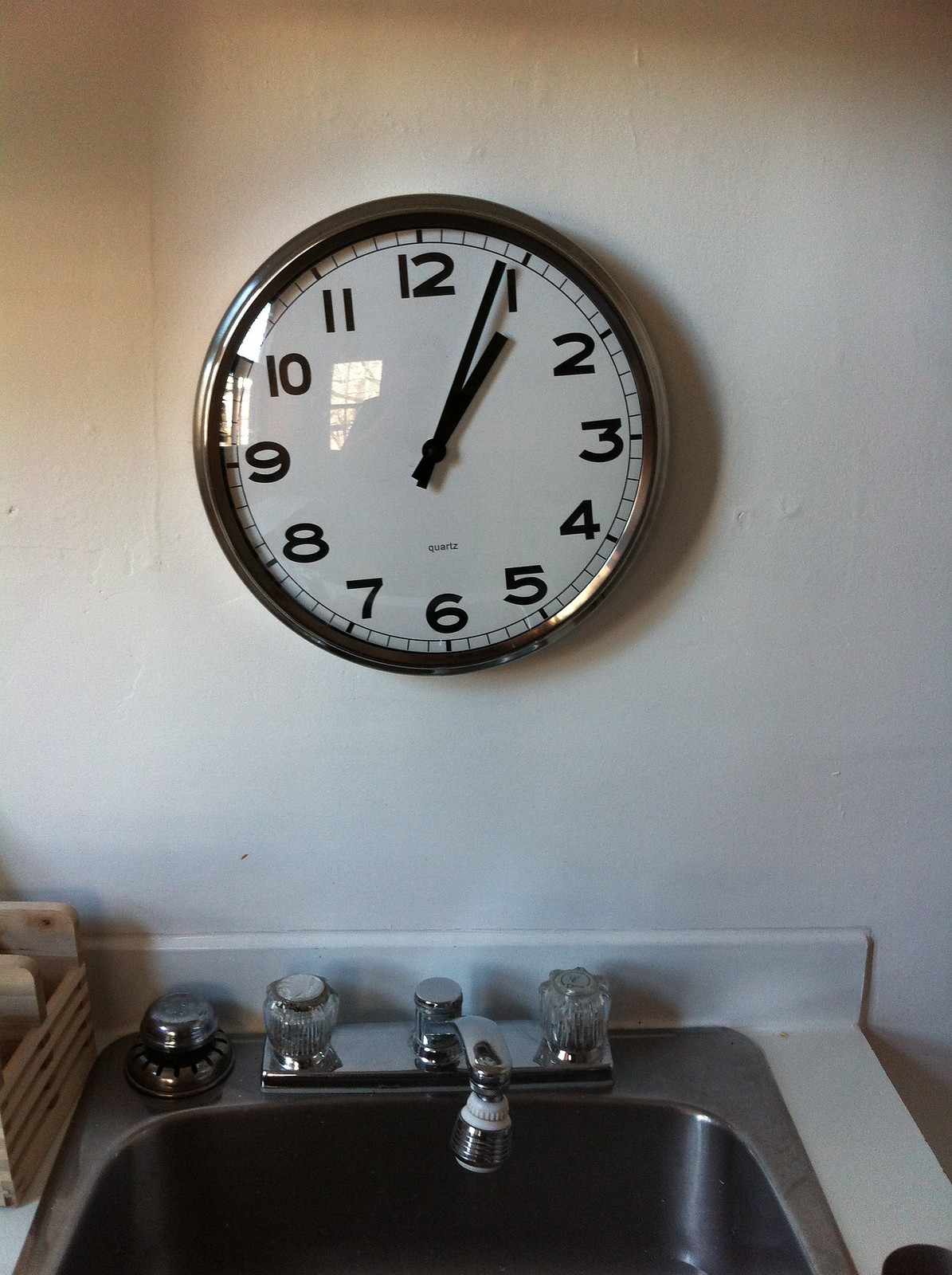This is a color photograph depicting a kitchen scene. On a white wall, a round wall clock with a black frame is prominently displayed. The clock features black numbers from 1 to 12 and black hands, with the hour hand pointing slightly past 1 and the minute hand precisely on top of 1, indicating a time of approximately 1:04. The clock's center is white, and the word "Quartz" is visible in small black letters above the number 6. Below the clock, there is a brushed aluminum sink with a single basin, inlaid in a white Formica countertop with a thin white backsplash. The sink has a silver, shiny faucet, complemented by clear plastic handles for hot and cold water. The strainer is removed and placed on the sink, which also features a light-colored wooden box on its left side. The photograph captures details such as a reflection in the clock, shadows on the wall, and a slight glare of light on the clock face.